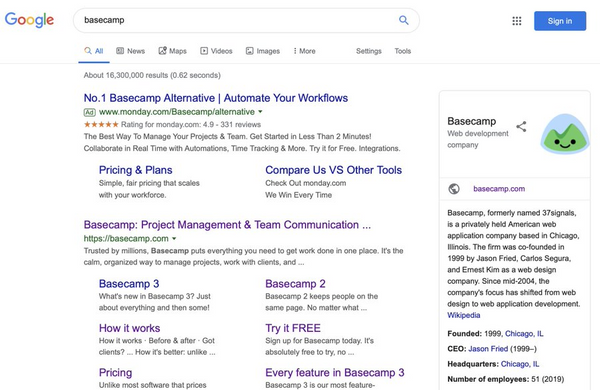A detailed depiction of a Google search results page dedicated to "Basecamp". Prominently displayed in the top left corner is the iconic Google logo, presented in its traditional blue, red, yellow, and green hues. The term "Basecamp" is entered within the central search bar, accompanied by a blue-highlighted magnifying glass icon on its right. Continuing rightward, a grid-like square icon and a "Sign In" prompt appear. The sign-in button is elongated and has a blue background.

Below the search bar, a navigation menu spans the width of the page, featuring the categories: All, News, Maps, Videos, Images, More, Settings, and Tools, each labeled with corresponding icons, except for Settings and Tools.

The first search result is labeled as an advertisement and garners the top listing, emphasizing "Basecamp alternative" followed by "Automate your workflows". A URL and a rating are displayed beneath, alongside links for "Pricing and plans" and a brief summary. Further links encourage a comparative analysis with other tools.

Subsequent sections include information on "Basecamp project management and team communication," details about "Basecamp 3," pricing options, and features available for trial. Additional segments focus on Basecamp's history, sharing options, and foundational details, providing a comprehensive overview of the software's offerings and functionality.